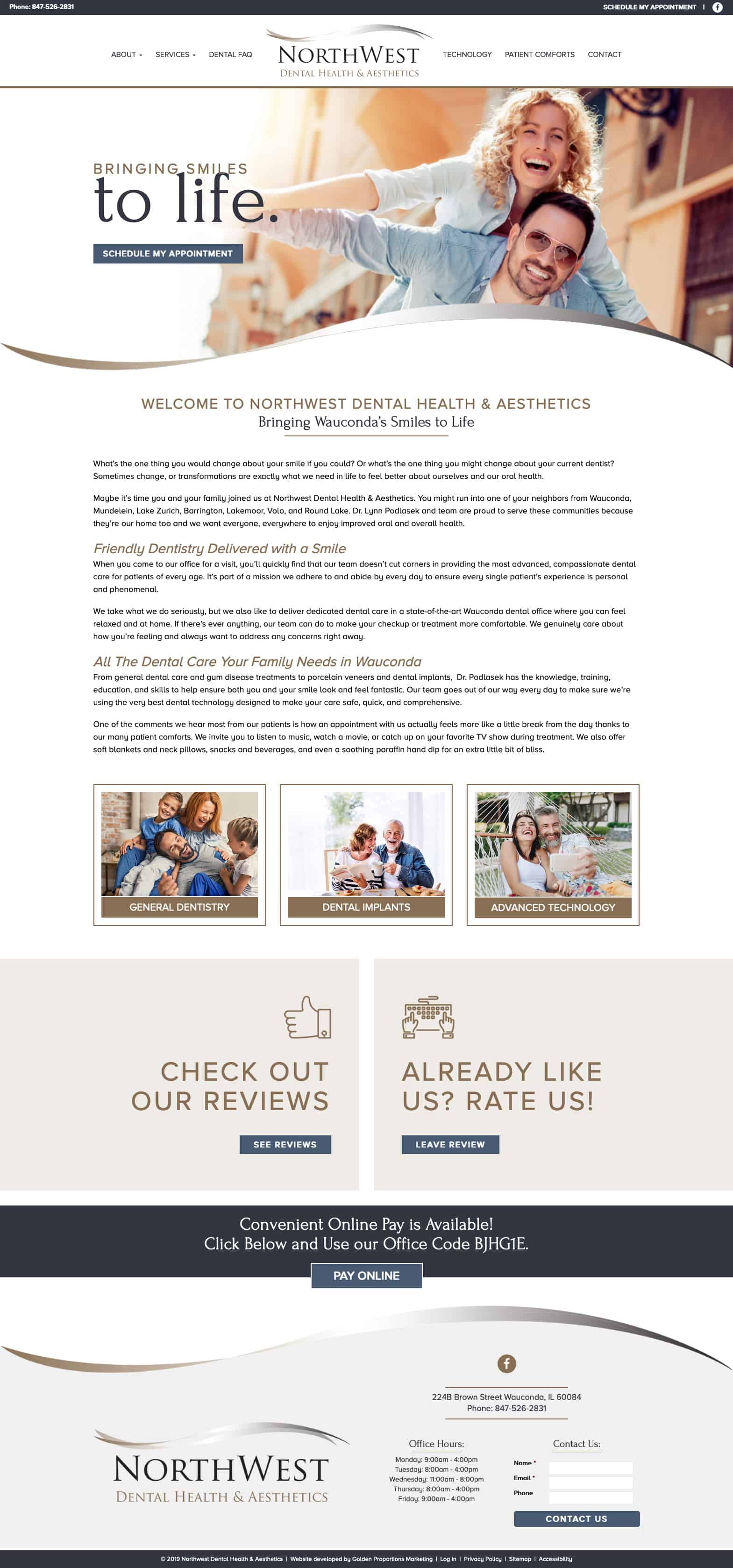Sure, here is a cleaned up and detailed caption for the image described:

---

On the Northwest website, the homepage features a prominent banner image at the top showcasing a cheerful couple engaged in a playful moment. The woman, smiling broadly, is playfully riding on the back of the man, who is also beaming with happiness, suggesting they are a couple, possibly significant others or spouses, enjoying their time together. Below the main image, there are several interactive tiles inviting users to "Check Out Our Reviews," "Already Like Us?" and "Rate Us." Additionally, three smaller thumbnail images are displayed, portraying various relationships: one image features a happy family, another captures an older couple embracing, and the last shows a younger couple in a loving embrace. The overall imagery and layout hint that this might be an insurance website, focusing on family, relationships, and well-being. Text on the page appears too small to read clearly, but the inviting photos and interactive elements suggest a welcoming and customer-oriented platform.

---